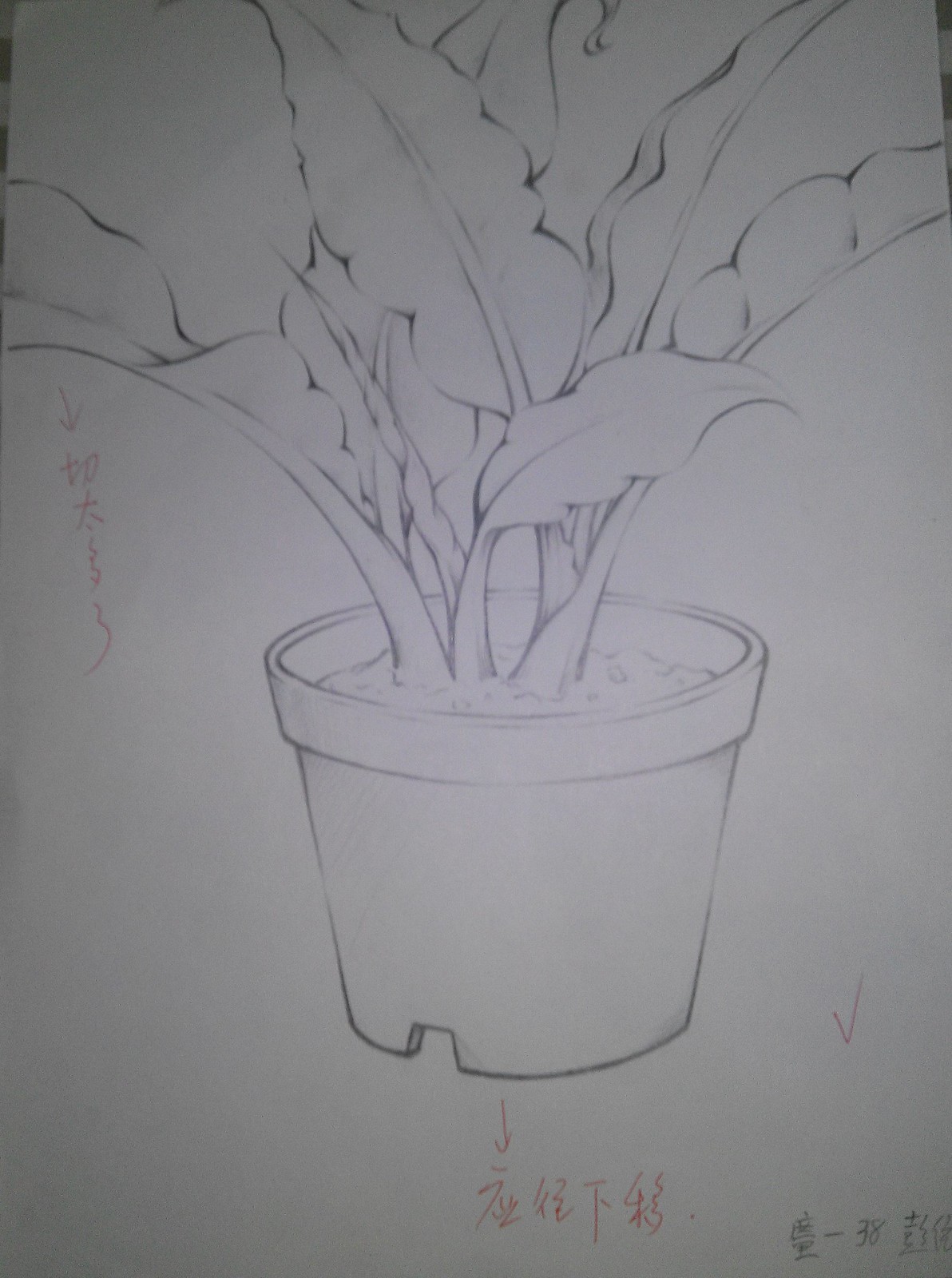This is a black and white drawing of a medium-sized plant in a moderately large pot. The plant features five to six visible leaflets, indicating its healthy growth. The illustration is complemented by text written in both red and black ink. The numeric figure '38' is prominently visible alongside additional writing in what appears to be Mandarin, though it is unclear whether it is in Simplified or Traditional script.